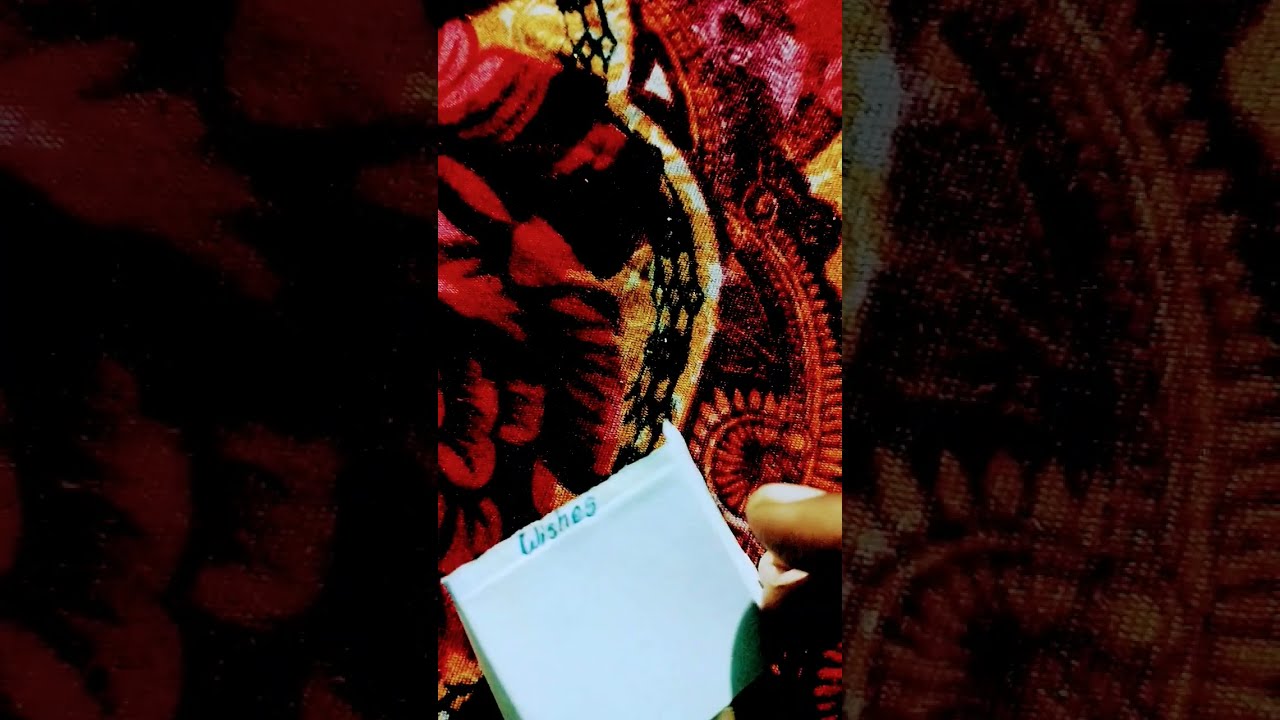The image displays a close-up view of a richly patterned floral fabric, which appears to be an oriental rug or cloth, showcasing intricate red flowers with black shadows, gold decorative circles, and red plant-like elements against its fabric. The entire background is adorned with these floral and circular motifs, rendered in various shades of red, green, brown, tan, yellow, black, gold, white, and pinkish hues. At the bottom center of the image lies a small white post-it note with the handwritten word "wishes" in blue ink. To the right, a hand with light brown or tan skin is visible, with two fingers pointing towards the note. The sides of the image are blurred, suggesting that this may be a screenshot captured from a mobile device, potentially on platforms like TikTok or Instagram.